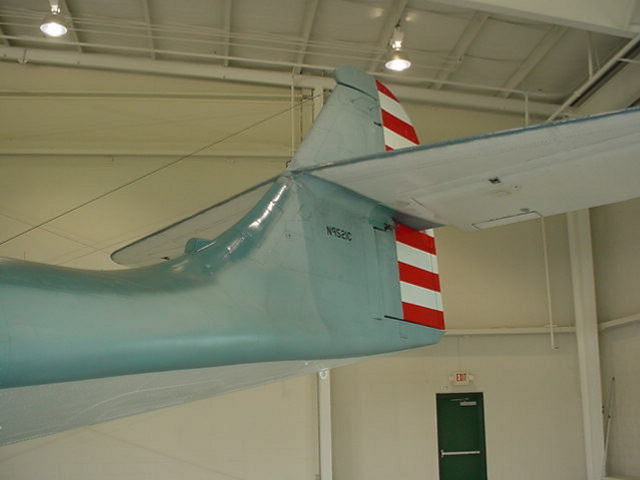This detailed image features an airplane inside a warehouse or hangar, captured from a 45-degree angle, focusing on the back quarter of the aircraft. The plane exhibits a striking color palette with a green fuselage and a tail adorned with red and white horizontal stripes on the vertical stabilizer. The horizontal wings, visible only from their underside, appear white. In the background, a black push door with an exit sign is mounted on a white wall. Overhead, two bright lights illuminate the scene, emphasizing the industrial setting. Additionally, the aircraft bears the identification number N95-2C.